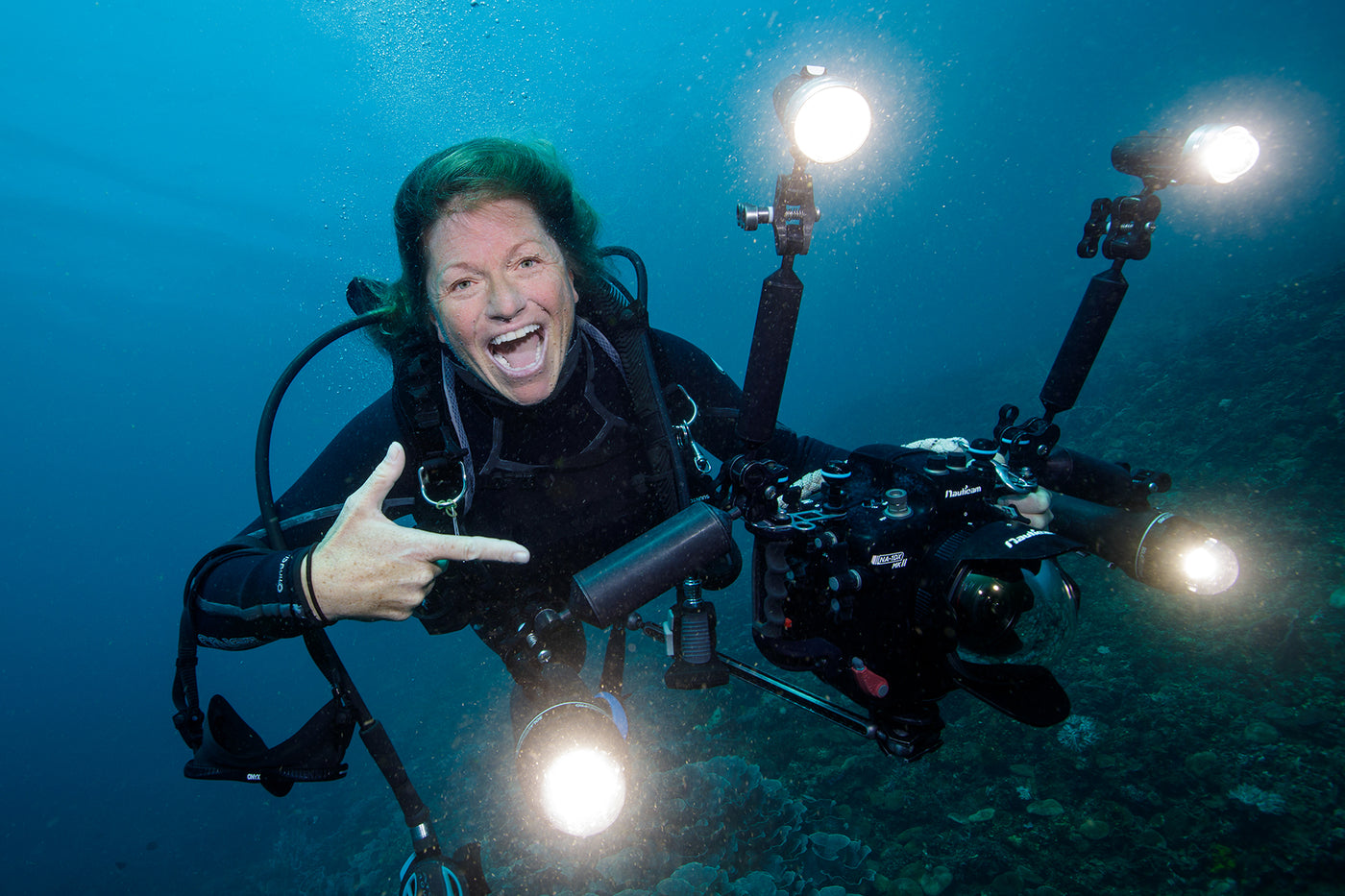This photograph captures a joyful female scuba diver underwater, presumably on the ocean floor. She has long, flowing blonde hair and is wearing an all-black wetsuit. Her goggles are draped over her arm, and her breathing apparatus is hanging off her side as she smiles widely with her mouth open, exuding happiness and excitement.

In her right hand, she holds a specialized underwater camera, characterized by its black body and a dome-shaped glass window over the lens. The camera is equipped with four cylindrical arms extending from its top and sides, each arm fitted with a bright LED light to illuminate the underwater scene. The woman points at the camera with her left hand, which is shaped in a playful gun gesture. Her enthusiasm and the high-tech equipment suggest she is engaged in underwater filming or photography.